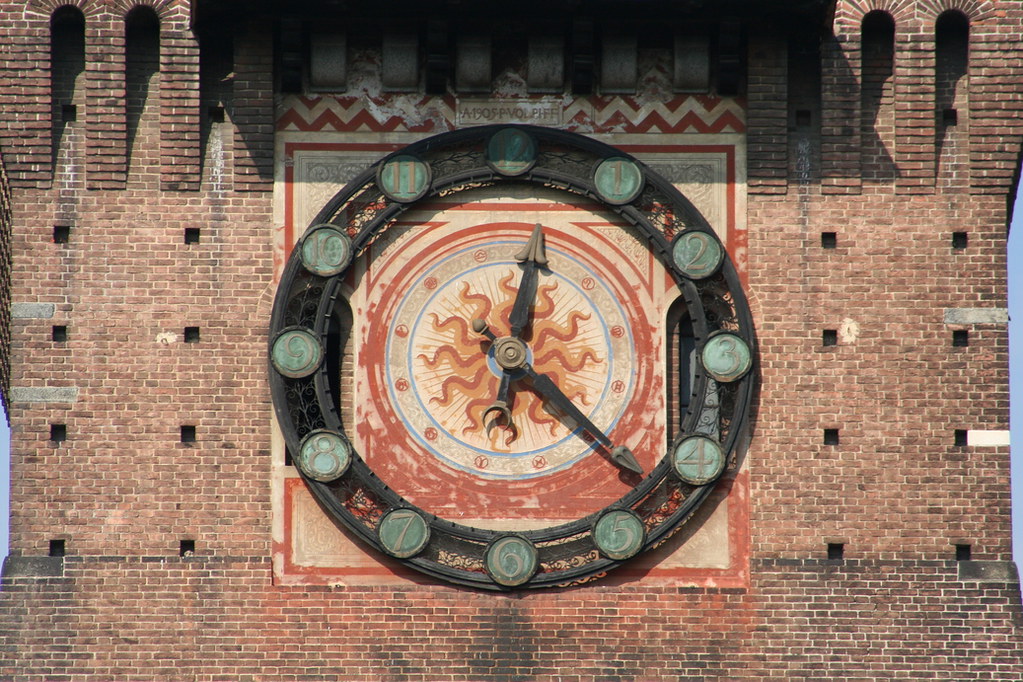This close-up photograph showcases the iconic clock tower of Sforza Castle in Milan, Italy. The clock, strikingly large in diameter, features bold numbers marking the hours, along with distinct hour and minute hands. Behind the hands, an intricate symbol resembling the sun, evocative of astrological designs, adds an artistic touch to the clock's face. The clock tower, integrated into the fortress-like structure of the castle, is constructed from red brick, lending a rich, historical aesthetic. Small peepholes punctuate the sides of the brick wall, hinting at the building's storied past. The image captures the architectural details with sharp clarity, offering a glimpse into the grandeur and age of this medieval fortress.